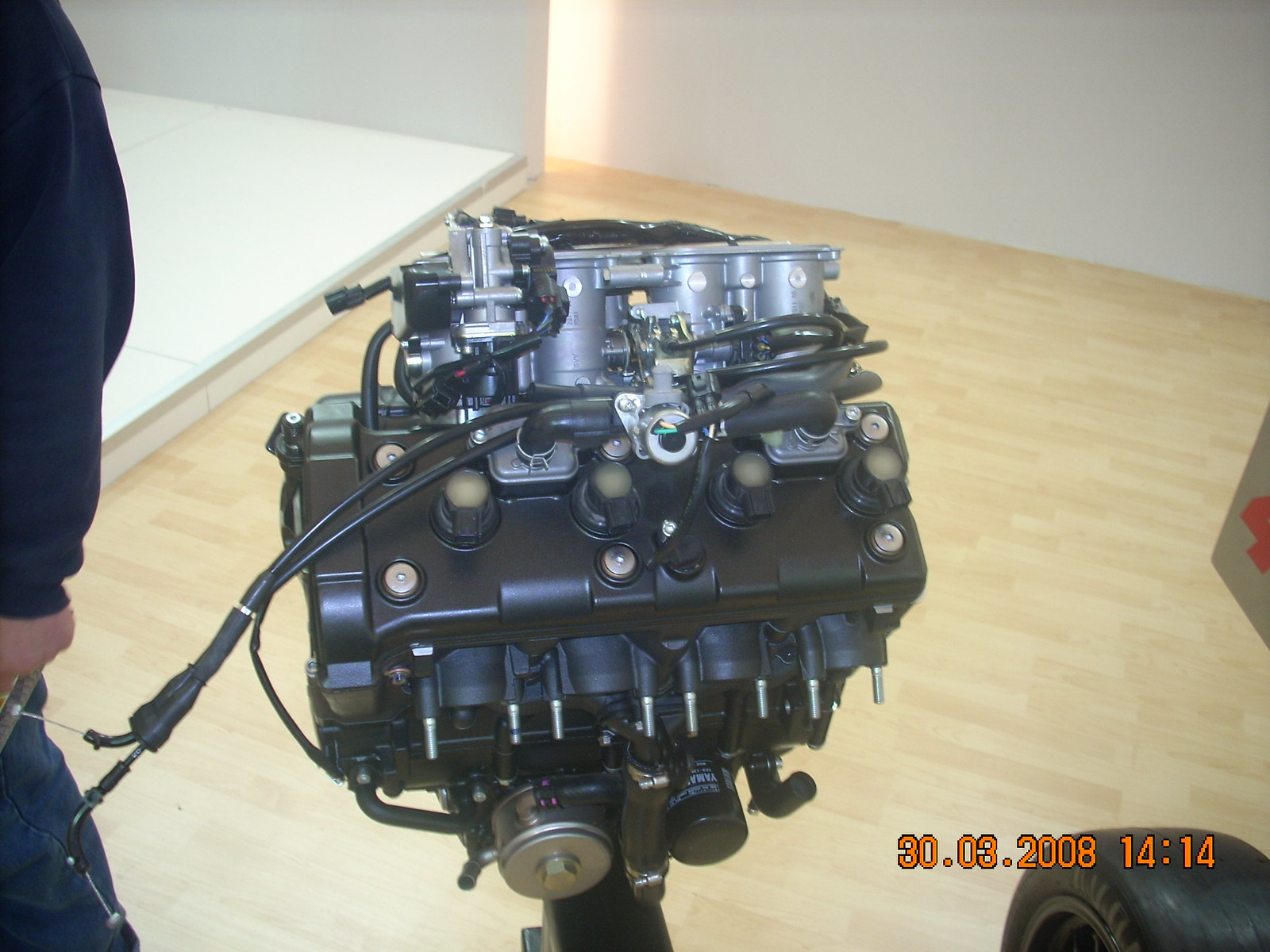The photograph captures a detailed display of a mechanical engine, situated on a light brown wooden floor with white walls in the background. The engine, primarily silver and black, features several wires and tubes protruding from its structure. The setup includes a raised white platform in the top left corner. The engine is the central focus of the image, highlighted by a person partially in the frame on the left side. The individual is wearing a long-sleeved blue shirt and blue jeans, with only their arm and the upper part of their leg visible. A black tire and white lettering are discernible near the bottom right corner, partially obscuring a timestamp in orange font with a black border, reading "30.03.2008 14:14".